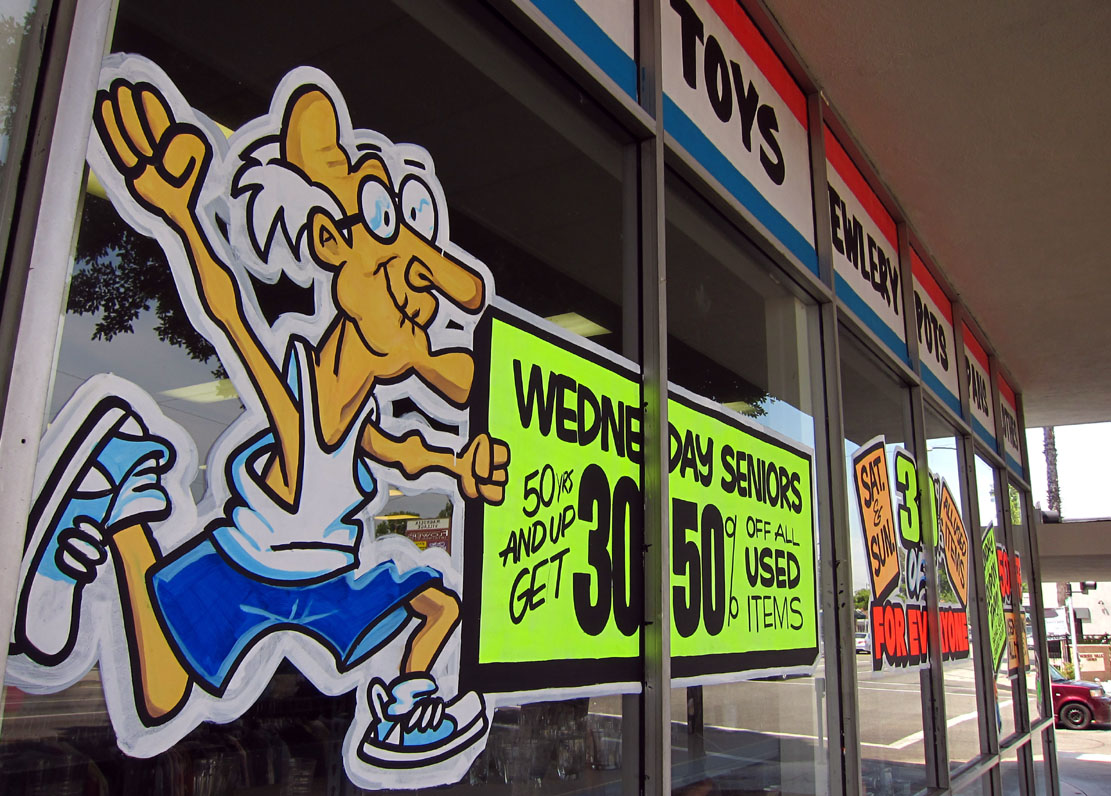In this vibrant photograph of a storefront window, the reflection of gray pavement from a nearby parking lot can be faintly seen. The top portion of the windows is adorned with a patriotic red, white, and blue stripe. Black lettering across the windows prominently announces the items sold within: "Toys," "Jewelry," "Pots," and "Pans."

Each window is decorated with bright, eye-catching designs. Notably, there is a cartoon-like, sticker-style image featuring an older, balding man wearing glasses, a white shirt, blue shorts, and blue-and-white sneakers. This illustration highlights a special offer: "Wednesday Seniors, 50 years and up, get 30 to 50% off all used items." Another window advertises a weekend promotion: "Saturday and Sunday 30% off for everyone sale." The combination of colors, text, and playful graphics creates an inviting and lively storefront display.